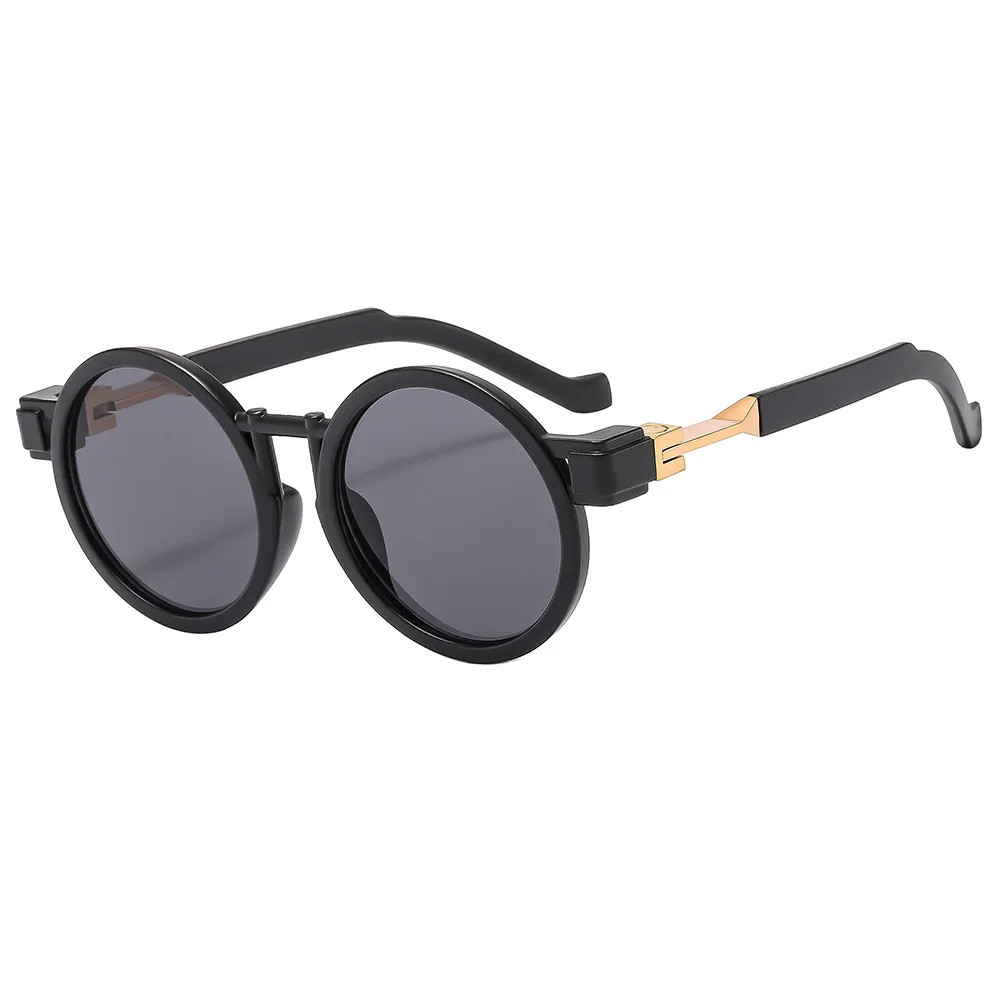The image features a pair of round, slightly tinted gray sunglasses with thick black frames. The lenses are somewhat transparent, offering a shaded view without being intensely dark. The glasses are depicted from a front view, slightly angled to one side, allowing a clear view of their entire form. Both earpieces, which are curved slightly downwards, are open and predominantly black with a striking copper or beige-colored hinge detail that adds a touch of retro flair to their modern design. The nose bridge, also black, has an unconventional square shape. The background of the photograph or realistic drawing is entirely white, giving the illusion that the sunglasses are suspended in mid-air.